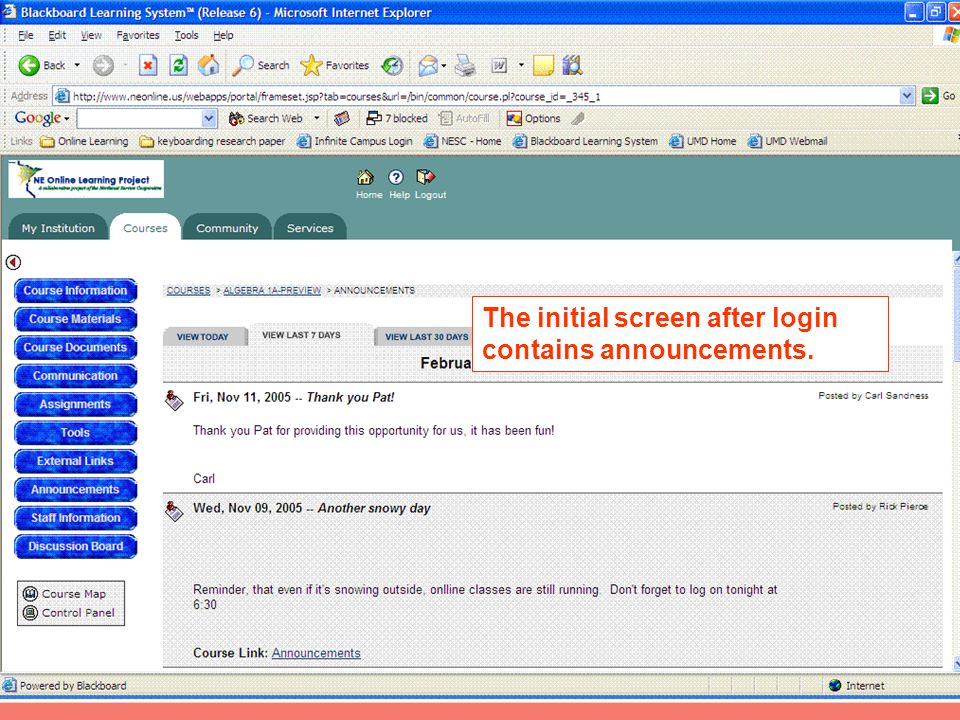The image displays a Google search set up on the browser's toolbar rather than the main search page, with no text entered into the search bar. At the top of the browser, the title reads "Blackboard Learning System - Microsoft Internet Explorer," indicating that the application is being accessed through this particular browser. Mid-page, prominently on the right side, a red box partially covers the content, highlighting an announcement on the initial login screen. The announcement mentions the "NE Online Learning Project," likely a segment of the institution’s online education platform. Different navigation tabs, including "My Institution," "Courses," "Community," and "Services," are visible. The "Courses" tab is currently active, displaying a filter bar on the left side of the screen for further navigation.